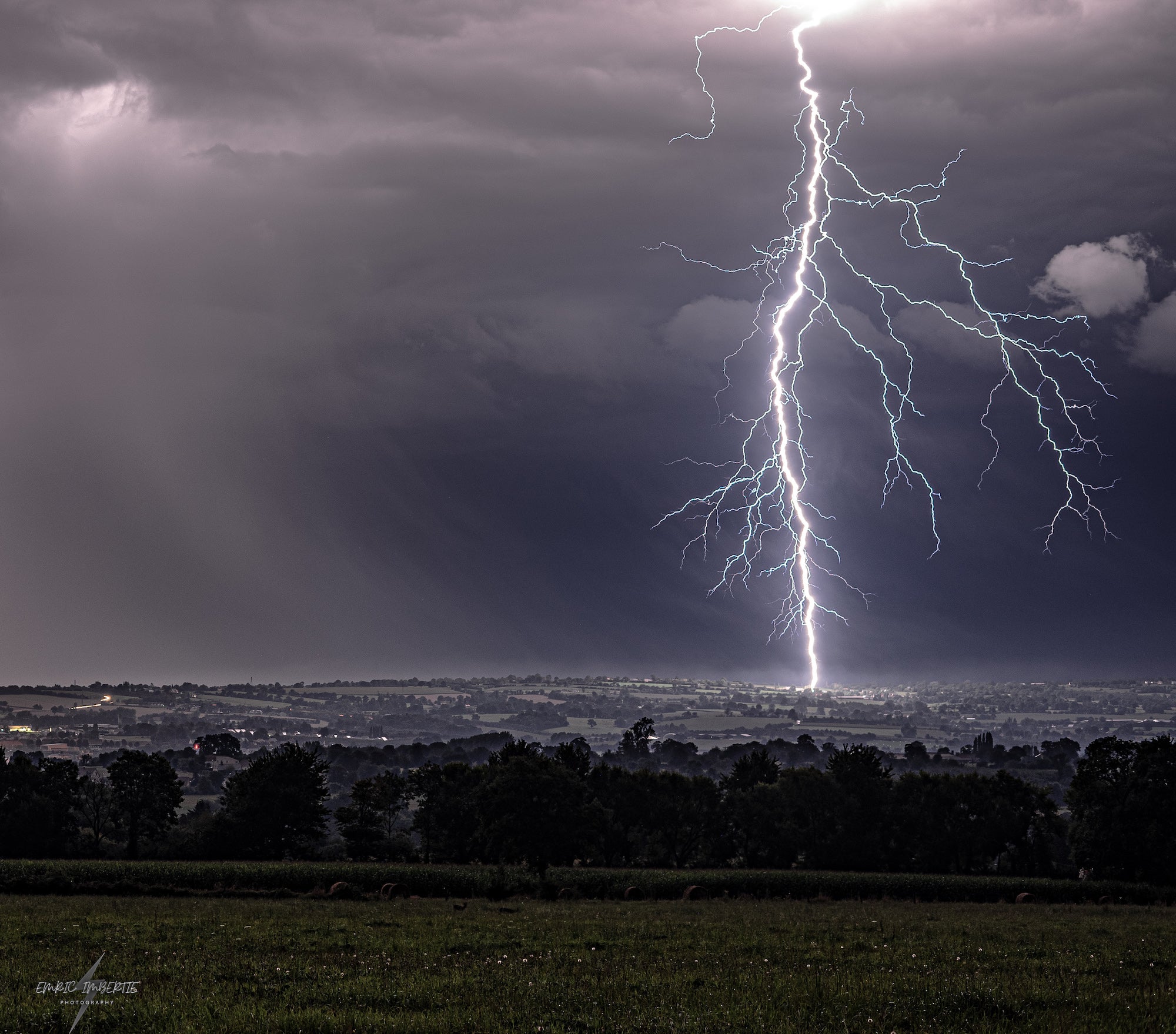This outdoor photograph, captured during a thunderstorm at night or dusk, presents a dramatic and imposing scene. The vast, flat landscape stretches out with a mix of trees and scattered houses, indicating a rural area. Dominating the right side of the image, a massive lightning strike spans from the top of the photograph down to the ground, with numerous branches radiating from the central bolt, illuminating the dark, cloud-filled sky. Sheets of rain can be seen pouring down from the clouds, adding to the atmosphere of the storm. The sky, which takes up most of the frame, is a deep, stormy gray, intermittently lit by both the lightning and a faint glow from the hidden moon. Below the sky, the terrain transitions from choppy ocean waters and a rocky beach to a grassy area with occasional bushes. The photograph also includes an unreadable name or title at the bottom left corner, and an inscription at the top that partially reads "exotic something photography," lending an air of mystery to this powerful and evocative scene.